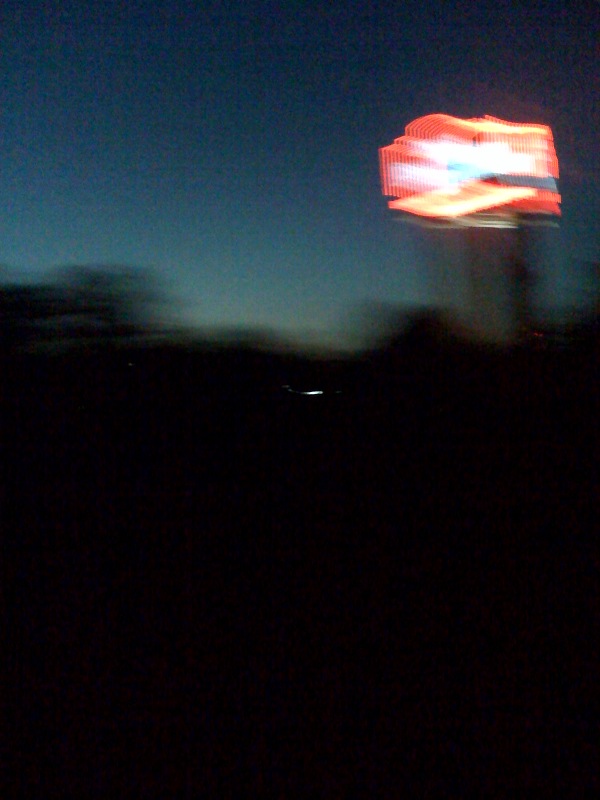This image appears to be a blurred photograph taken during the early evening or late afternoon. The lower half of the image is almost entirely obscured by darkness, rendering it a solid black. On the horizon towards the left side, there is a faint and indistinct outline of a tree. The sky above is a gradient of blues, with a darker blue hue dominating the top portion and gradually lightening as it reaches the horizon, suggesting the onset of dusk.

On the right side of the image, there is a straight, vertical post that appears to be gray. Attached to this post is a brightly colored rectangular sign. The sign features a bold red border and a design composed of various colors: predominantly white, with a blue horizontal stripe and some scattered yellow elements. Despite the blurriness, the vivid colors of the sign stand out against the dimming backdrop.